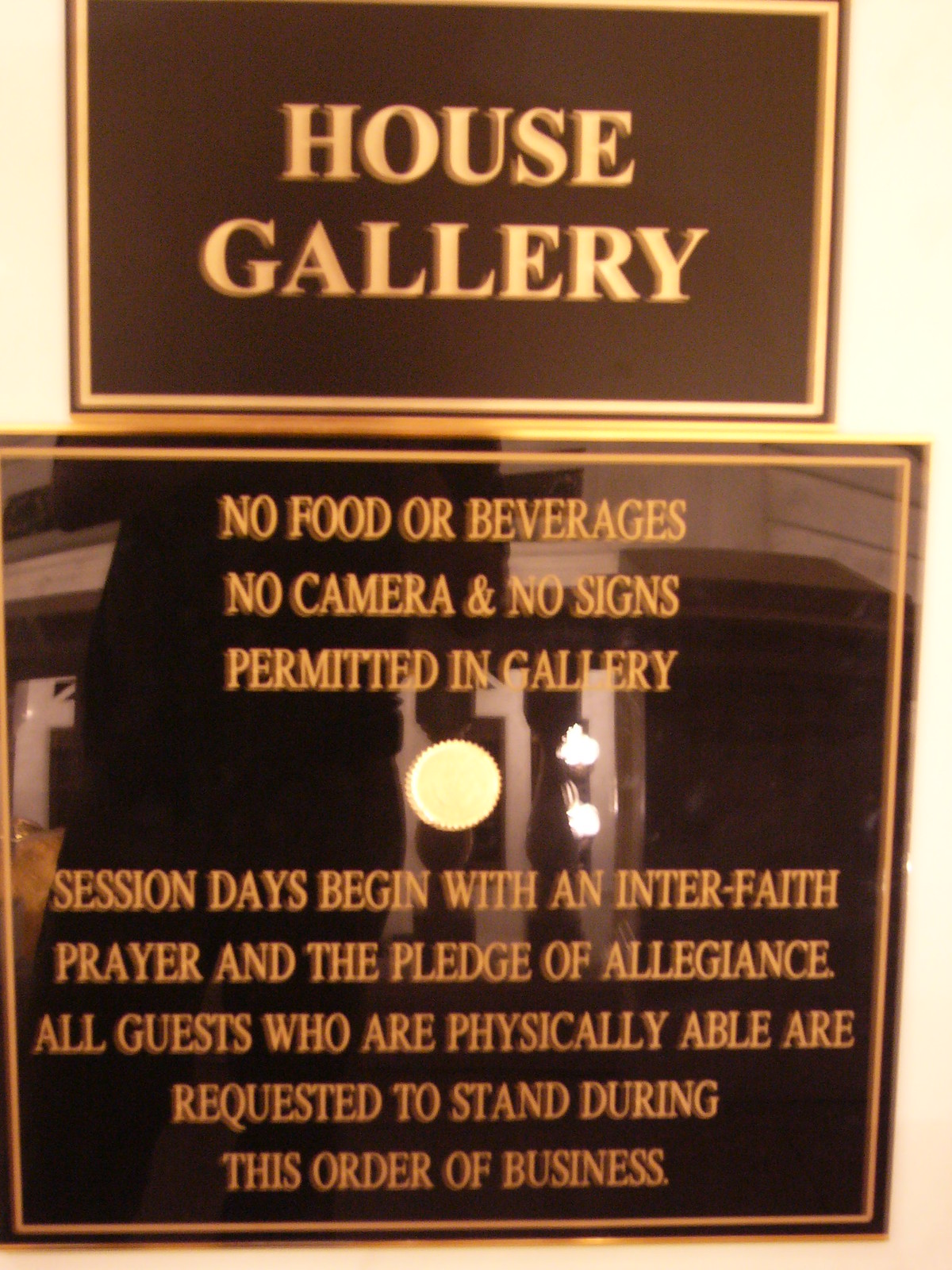The image captures a slightly blurry rectangular portrait of two plaques mounted on a cream-colored wall. Both plaques have a dark brown background with golden borders and gold lettering. The smaller, rectangular plaque at the top is partly cut off but prominently displays "HOUSE GALLERY" in all caps. Below it, a larger, square plaque lists several rules in gold text: "NO FOOD OR BEVERAGES, NO CAMERAS, AND NO SIGNS PERMITTED IN GALLERY." Further down on this plaque, it details that "SESSION DAYS BEGIN WITH AN INTERFAITH PRAYER AND THE PLEDGE OF ALLEGIANCE. ALL GUESTS WHO ARE PHYSICALLY ABLE ARE REQUESTED TO STAND DURING THIS ORDER OF BUSINESS." The plaques have a shiny surface reflecting parts of the room, including what appears to be banisters and possibly the person taking the photograph, giving the image a mirror-like quality.